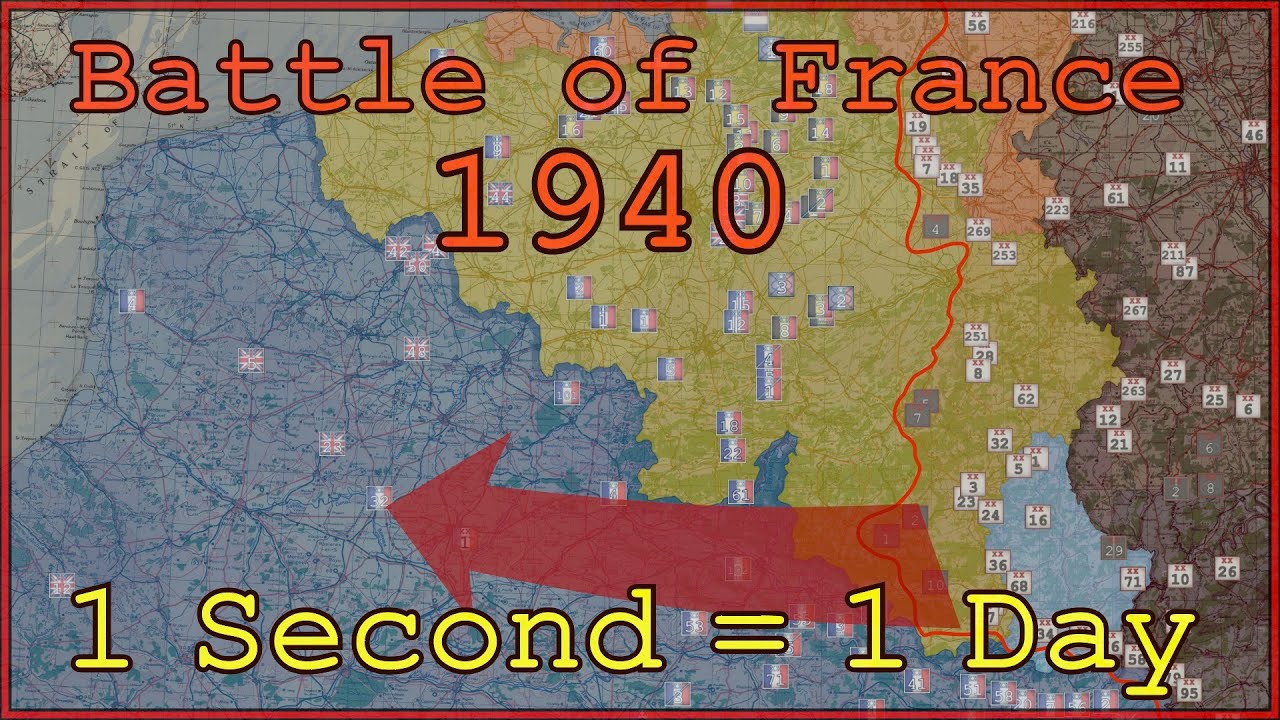This detailed color map of Europe during World War II serves as a graphical representation of the Battle of France in 1940. Overlaying the top of the image in large, red text outlined in black, is the title "Battle of France 1940." At the bottom, a legend in yellow text with a black outline states, "1 second equals 1 day." The map prominently focuses on Western Europe, with distinct sections colored to represent different territories: France is shaded in blue, Germany in light green, and a portion of the Soviet Union in brown. Scattered across the map are national flags of France and Britain, possibly marking significant battle locations or key events. A strikingly large red arrow swoops from southern Germany into the heart of France, indicating the primary direction of the German invasion. The entire image has a transparent red border that adds to the dramatic and intense presentation of the historical event.